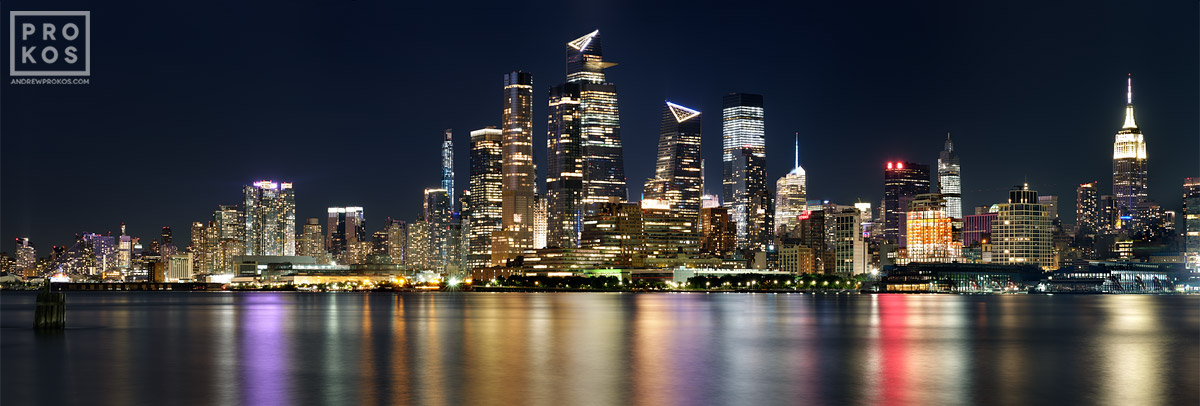This image features a stunning cityscape view of a modern metropolis at night, with an expansive horizontal panorama that stretches about two and a half to three times its vertical height. In the foreground, a serene river or lake reflects the city’s vibrant lights in hues of white, red, blue, purple, and even some green. The night sky is clear, devoid of clouds, framing the illuminated skyline beautifully.

Dominating the scene, a series of skyscrapers, with the tallest structures centralized, create an impressive silhouette against the night. As the gaze moves to the right, the buildings transition to slightly shorter, though still imposing heights. To the left of the tallest cluster, a possibly discernible bridge adds an element of structure, enhancing the urban composition. 

In the top left corner of the image, a watermark reads "Prokos" with the letters "P-R-O" stacked atop "K-O-S," distinctive within a gray box. Subtler details like the potential outlines of ships or boats near the buildings, and the reflection of colored lights on the water, add depth and intrigue to the city's nocturnal charm.